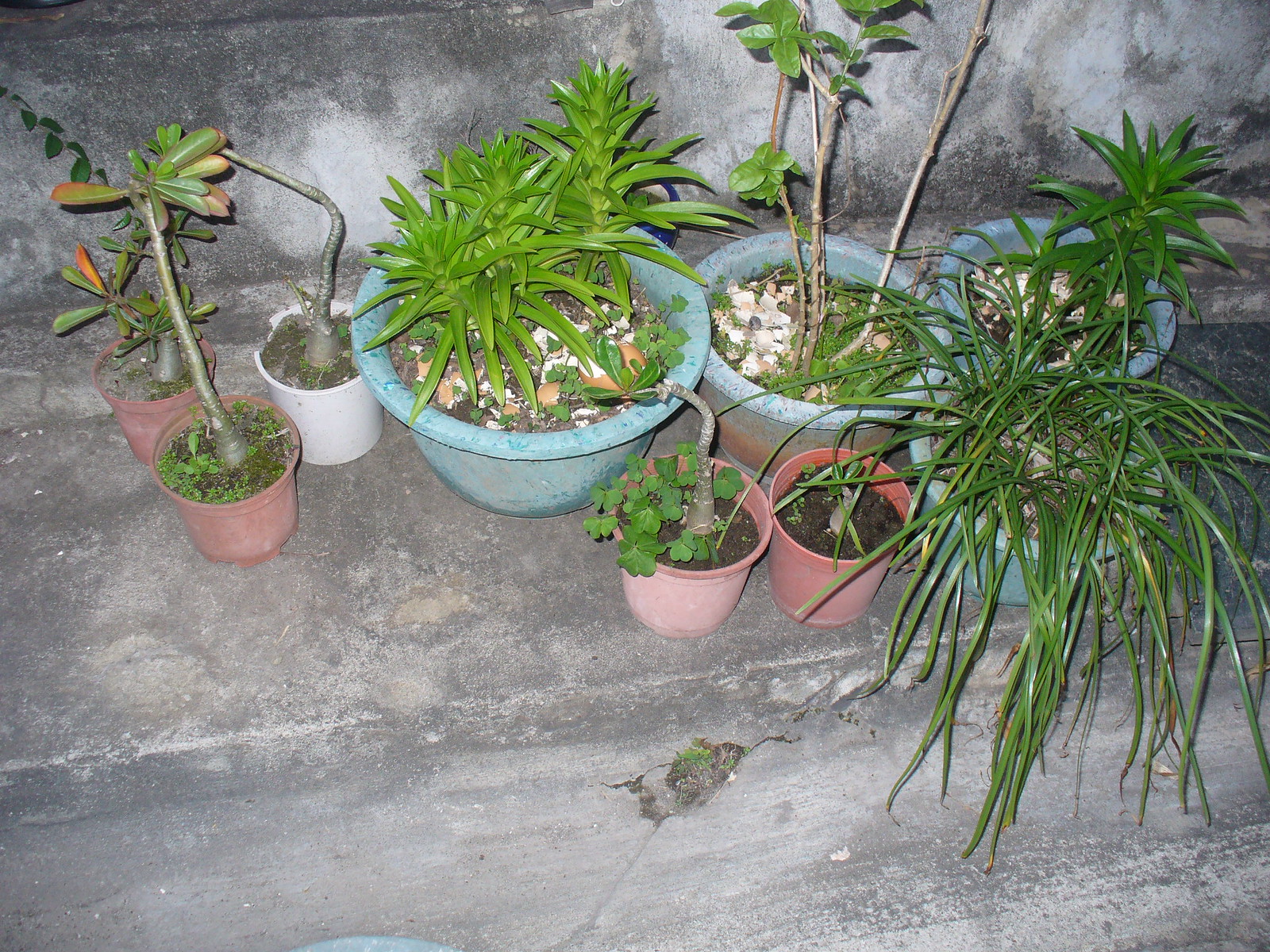This outdoor color photograph captures a collection of nine potted plants arranged on a weathered, mottled concrete surface next to a concrete wall. The concrete appears old and faded with shades of white, brown, and gray. The plants are all placed on the same step-like area, contributing to a cohesive, albeit slightly cluttered, feel. The majority of the pots are larger and blue, positioned towards the back, while the smaller pots, including a couple of reddish-clay and one white pot, are positioned towards the front. Among these are three smaller pots on the left, two of which are red and possibly ceramic or plastic, containing jade plants, and a white pot also likely containing a jade plant. Towards the center is a notable blue pot with green plants boasting narrow leaves. To the right is another blue pot with three slender brown stalks. Adjacent is a similar blue pot with long slender green leaves extending into the foreground. Near these are two smaller pots with scant plants, mainly showing dirt. Other varieties include plants with long, thinner leaves, likely spider plants, some possibly clover, and a few with the appearance of small trees, growing upwards. This eclectic mix of plants, though somewhat bedraggled, is an earnest attempt at adding greenery to the home environment.